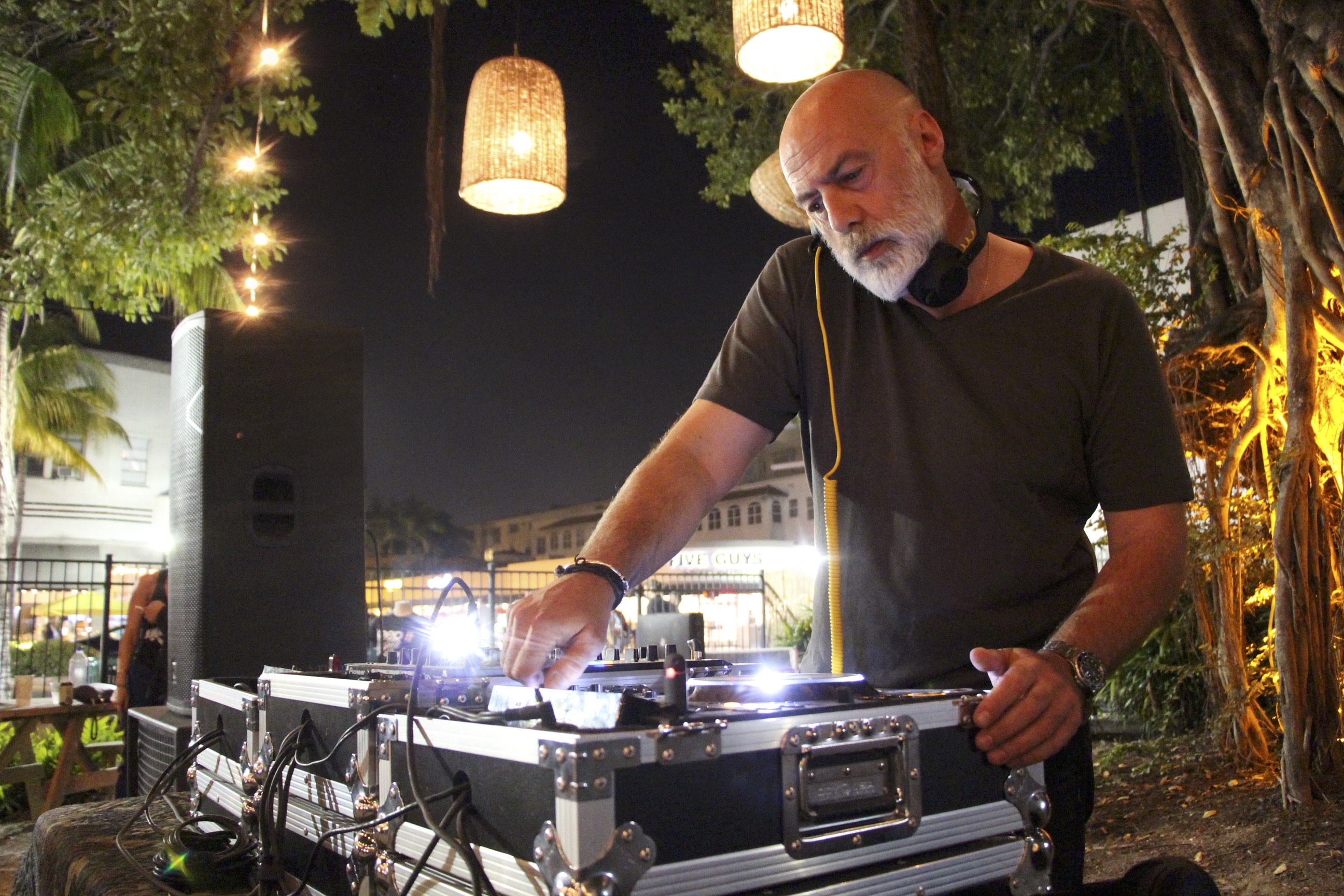In this vibrant nighttime color photograph, we see a DJ engrossed in his equipment, standing in an outdoor urban setting under a tree adorned with golden lights. The man, a Caucasian male with a bald head and a gray beard, is wearing a short-sleeved, dark-colored V-neck t-shirt and a watch. Resting around his neck are black headphones with a distinctive yellow cord connecting to his sophisticated DJ equipment. The equipment, appearing in sleek black and silver, resembles several stacked travel cases with various black cords snaking out. The man's hands are actively engaged, turning knobs and managing his setup, which sits atop a table covered by a tablecloth. The backdrop reveals a dark, night sky with illuminated buildings, suggesting a lively city atmosphere. Nearby, thin branches sprout from the ground, adding a touch of natural ambiance enhanced by twinkling lights wrapped around the tree trunk and hanging from above. Surrounding him is a black metal fence, framing the scene. Two additional lights shine down from above, providing ample illumination for his performance.